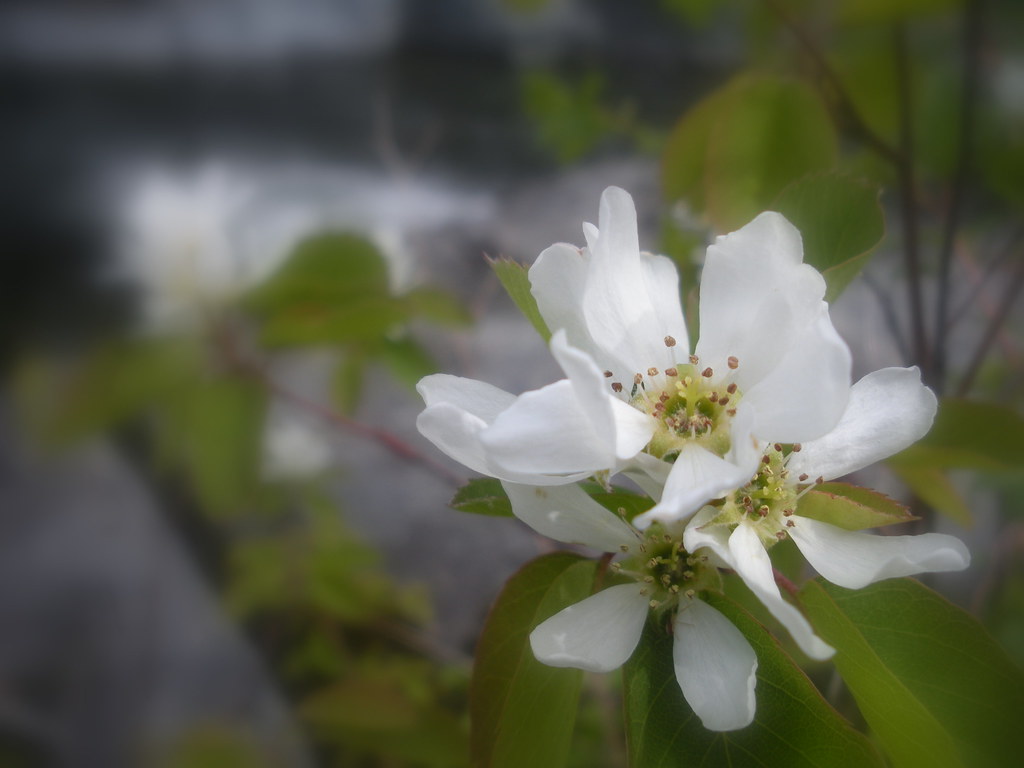This photograph captures an elegant white flower in a macro setting, sharply in focus against a blurred and muted background. The primary subject, occupying the lower right quadrant of the frame, displays a cluster of three to four blossoms on one branch. The flower, possibly resembling a lily, features pristine white petals and a central cluster of pistils or seeds. Green leaves surround the blossoms, though they, too, are slightly out of focus, contributing to the photograph's overall soft and whimsical aesthetic. The surrounding flowers and foliage are also present but rendered indistinct by the shallow depth of field and a potential filtering effect, creating a dreamy, almost satin-like texture in the blurred areas. The lighting suggests an overcast day, with the subdued greenery and muted tones enhancing the serene and delicate beauty of the scene.